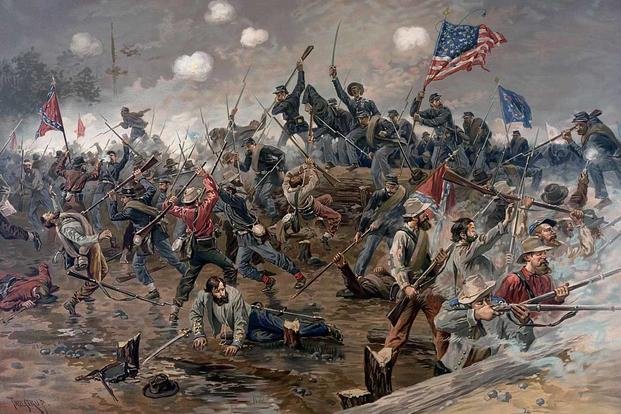This painting depicts a chaotic and fierce battle scene, likely from the American Civil War. Men, in varied uniforms signifying both Union and Confederate soldiers, are embroiled in violent combat. Many hold long rifles and swords, while some are actively shooting, evidenced by the smoke clouds filling the sky. In the background, an American flag is being held high, symbolizing a claim of victory, juxtaposed with another figure defiantly waving a Confederate flag, highlighting the ongoing struggle for dominance. The scene is punctuated by wounded soldiers lying on the ground, attempting to crawl away amidst the tumult. The smoky, cloudy sky adds a somber, dramatic backdrop to the turmoil of the battlefield, with the violence and confusion vividly portrayed through the soldiers' intense expressions and actions.